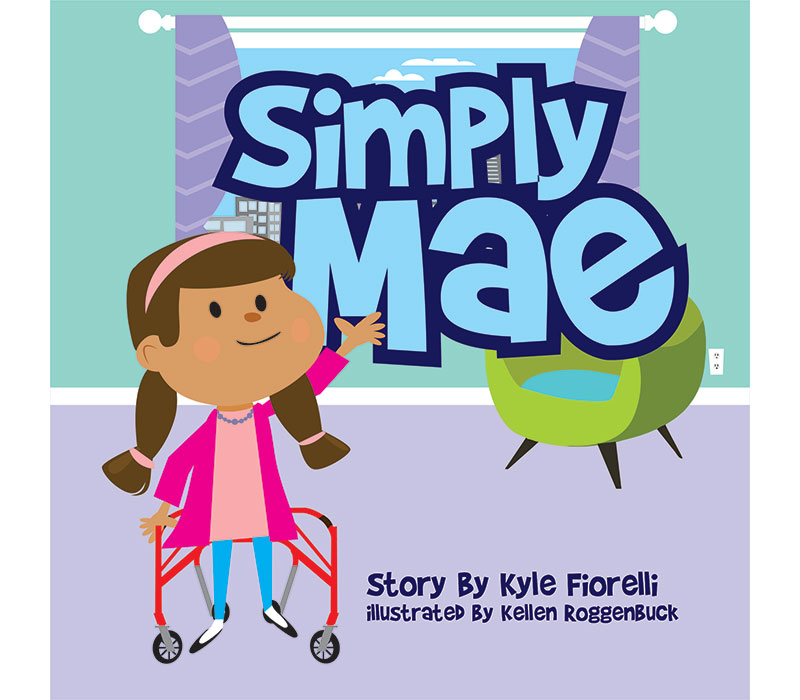This vibrant children's book cover, titled "Simply Mae," showcases a charming cartoon girl standing slightly to the left. The title "Simply MAE," spelled out in alternating black, dark blue, and baby blue letters, hovers above her head. The girl has dark brown hair styled into pigtails secured with pink barrettes and is adorned with a pink headband. She is warmly dressed in a pink jacket over a lighter pink shirt, complete with a purple necklace, blue jeans, white socks, and black ballerina flats. Her right hand is gripping a red walker that assists her in walking, while her left hand is joyfully extended into the air. Her expression is cheerful, with a beaming smile on her face. 

The backdrop features a large window with open purple curtains, revealing a clear blue sky and distant buildings. To the right, there's a modern lime green chair with a baby blue seat cushion and brown legs. The room has light blue walls and purple carpeting. Below the image, the text reads, "Story by Carl Fiorelli, illustrated by Kellen Roggenbuck."